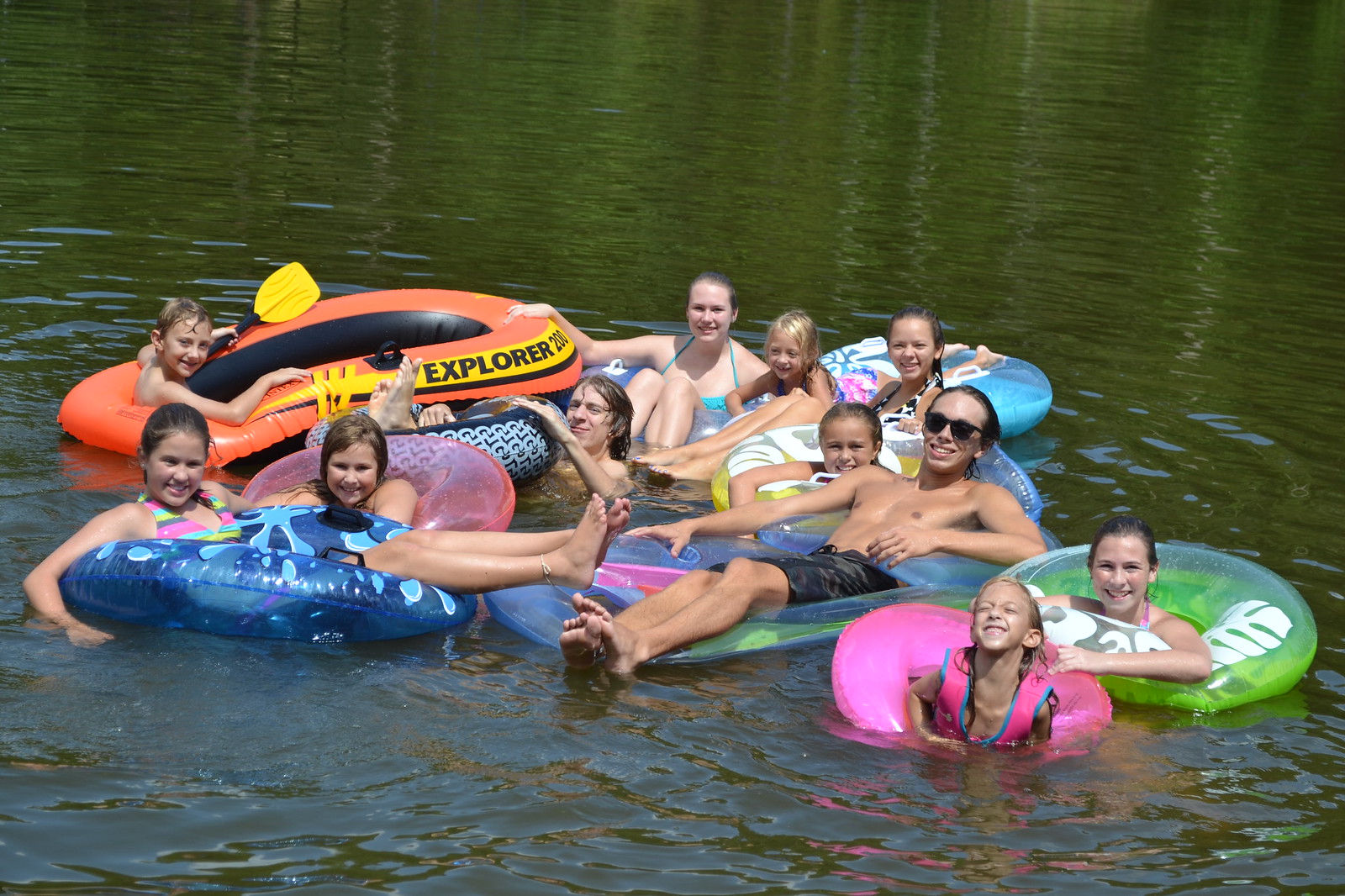In the vibrant photo captured at a greenish rippled lake, eleven kids, all seemingly under the age of 15, are enjoying a playful day on the water. They are comfortably nestled in an array of colorful inner tubes, ranging from warm hues of pink, green, and blue to a translucent top with a neon green bottom. Each child, clad in bathing suits, beams at the camera, their youthful joy evident. One boy stands out, sporting sunglasses and occupying an orange and black raft marked "Explorer 200," vividly adorned with an orange paddle. Another notable detail is a girl in the lower right corner who is seated in a pink inner tube and wears a life jacket. Amidst the sea of vibrant inflatables and youthful exuberance, two kids can be seen splashing directly in the water without flotation devices. The scene encompasses the bottom right corner to the middle left of the frame, a harmonious mix of colors including pinks, greens, blues, blacks, yellows, and tans, capturing a lively summer moment.